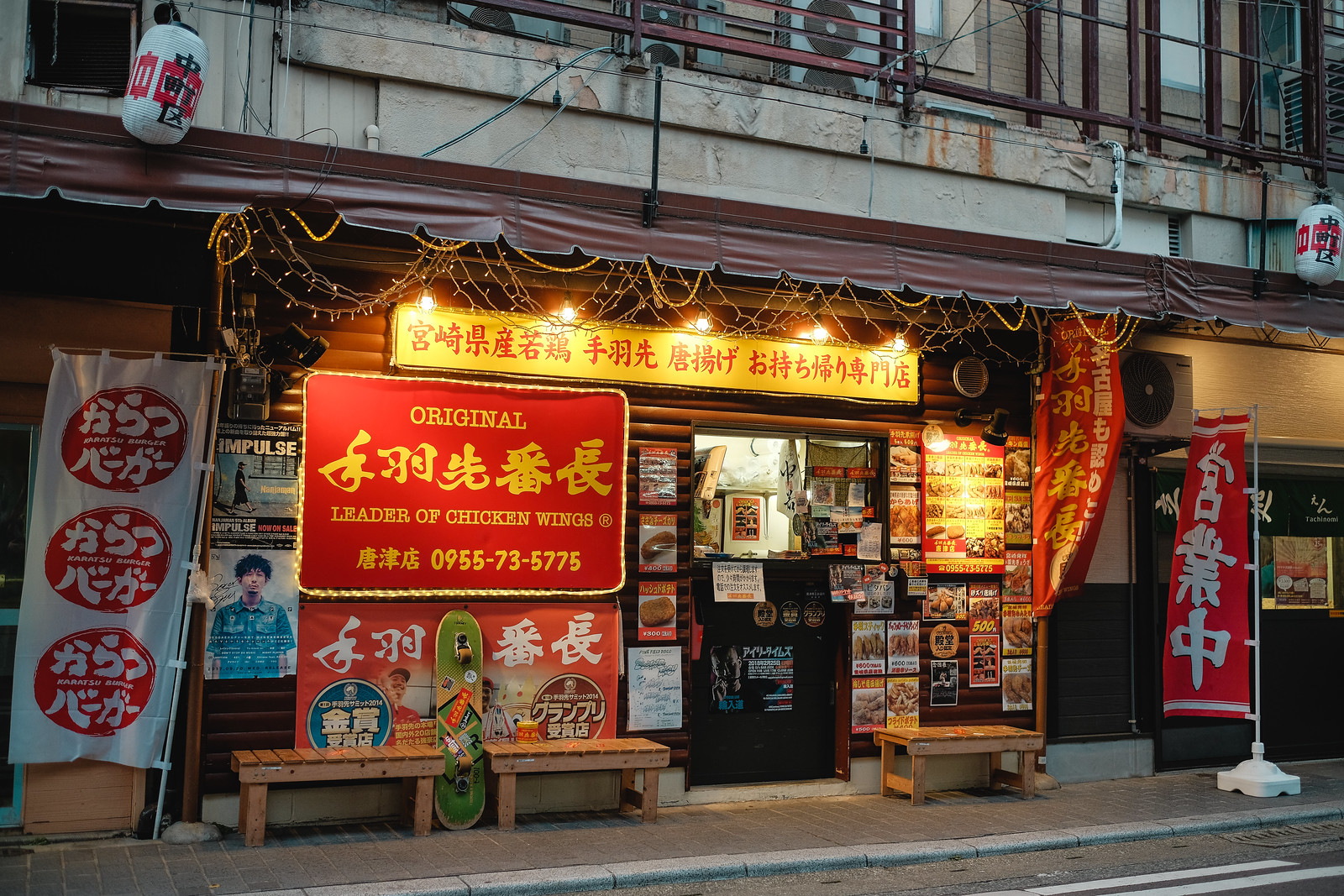This colorful and vibrant storefront, likely located in Chinatown, depicts the façade of a Chinese restaurant or store specializing in chicken wings. The upper eighth of the image showcases the cement building with windows and possibly a fan. The storefront beneath features a prominent yellow banner with red Chinese symbols stretching horizontally. To the left, there's a large red sign with yellow text reading "Original Leader of Chicken Wings," accompanied by a phone number: 0955-73-5775, and more Chinese characters. 

Below the sign, on the sidewalk, three red circles stacked vertically enclose more Chinese symbols. An orange sign featuring Chinese characters and a green cucumber motif peeks up from the sidewalk. Wooden benches are positioned in front of the storefront, providing seating for patrons. The middle of the image shows a black door adorned with small posters, possibly advertisements or a menu showcasing various food items. To the far right, a vertical red banner with white Chinese lettering hangs next to another door. The storefront is brightly lit, filled with images of food, and exudes a bustling, welcoming atmosphere.